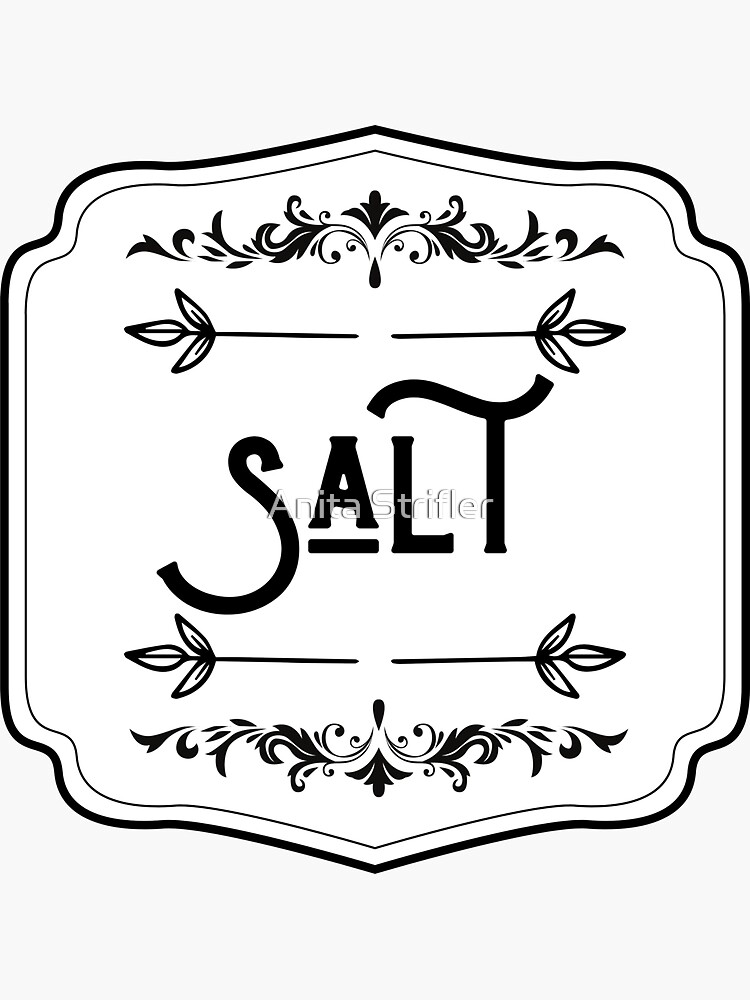This image depicts a vintage-style black and white label designed for a salt container. The label, set against a white background, features a prominent, thick black border with a thinner black line just inside it, creating a layered frame effect. The word "salt" is written in large, bold black letters at the center of the label. Above and below this central text, there are symmetrical floral designs: each features one flower bud with two leaves extending to the left and to the right. The overall design is evocative of 1920s style, complete with intricate etchings and flourishes that add a classic touch.